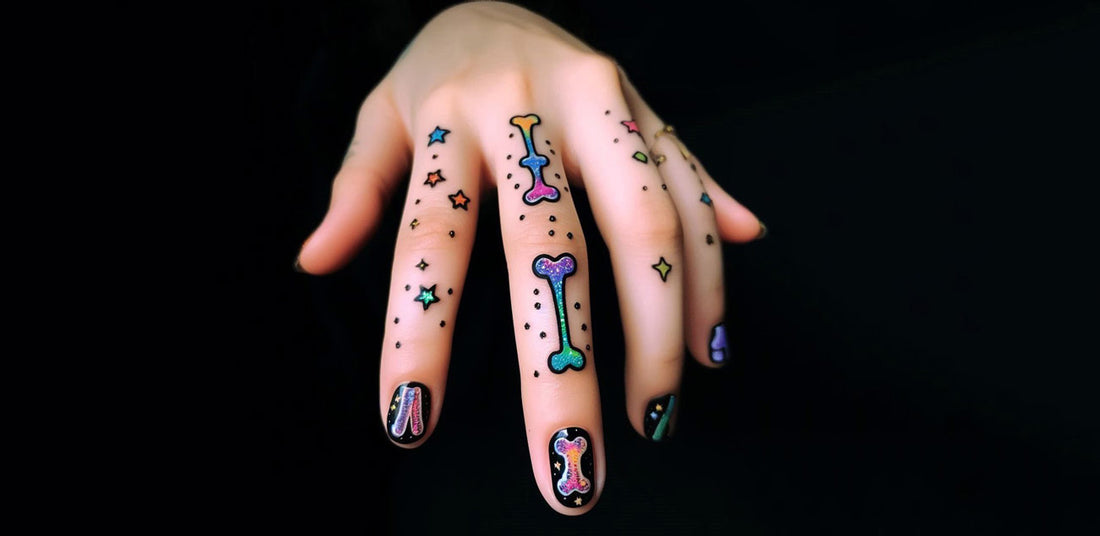This is a close-up photograph of a woman's left hand, positioned centrally against a black background, creating a striking contrast. The hand, with a pinkish flesh tone, features intricately detailed and colorful designs on both the fingernails and fingers themselves. Her fingernails are painted black and adorned with various vibrant designs, including stars and bones. Specifically, the index finger displays a couple of detailed stripes—one purple and the other reddish—surrounded by stars in blue, green, yellow, and red. The middle finger showcases a bone design that transitions fluidly from yellow at the top to blue, then pink, with dots and additional stars around it. Both the middle figurine's fingertip and fingernail continue this skeletal theme. The remaining fingers also exhibit intricate designs and stars, contributing to the overall artistic display. The hand appears to be a showpiece, enhanced with glitter and polish that enhances the visual appeal of the nails and the skin, showcasing a wide spectrum of colors including black, beige, pink, purple, green, blue, red, yellow, and orange.